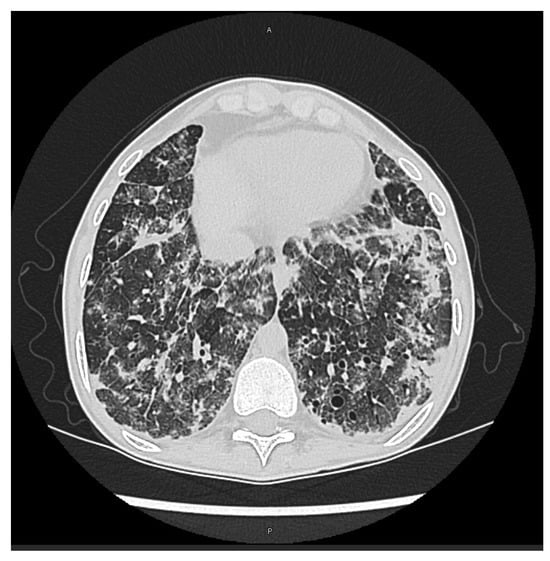The image is a detailed, monochromatic illustration resembling a medical x-ray or photocopy. Dominated by black, gray, and white tones with no accompanying text, the composition showcases a large, circular white ring set against a dark background, evoking the impression of a modern art piece. Surrounding the circle are rib-like cross sections extending vertically on each side, with five oblong white ovals interspersed among them. The interior of the circle features a dark, textured area with scattered white markings, reminiscent of paint splatter. At the bottom right, two prominent bone-like structures, likely representing parts of the spine, can be observed. Around the edges of the image, squiggly lines and white bands add to the complexity, possibly symbolizing cellular elements. The overall presentation suggests a cross-sectional view of an anatomical structure, perhaps the abdomen, seen through an artistic lens.